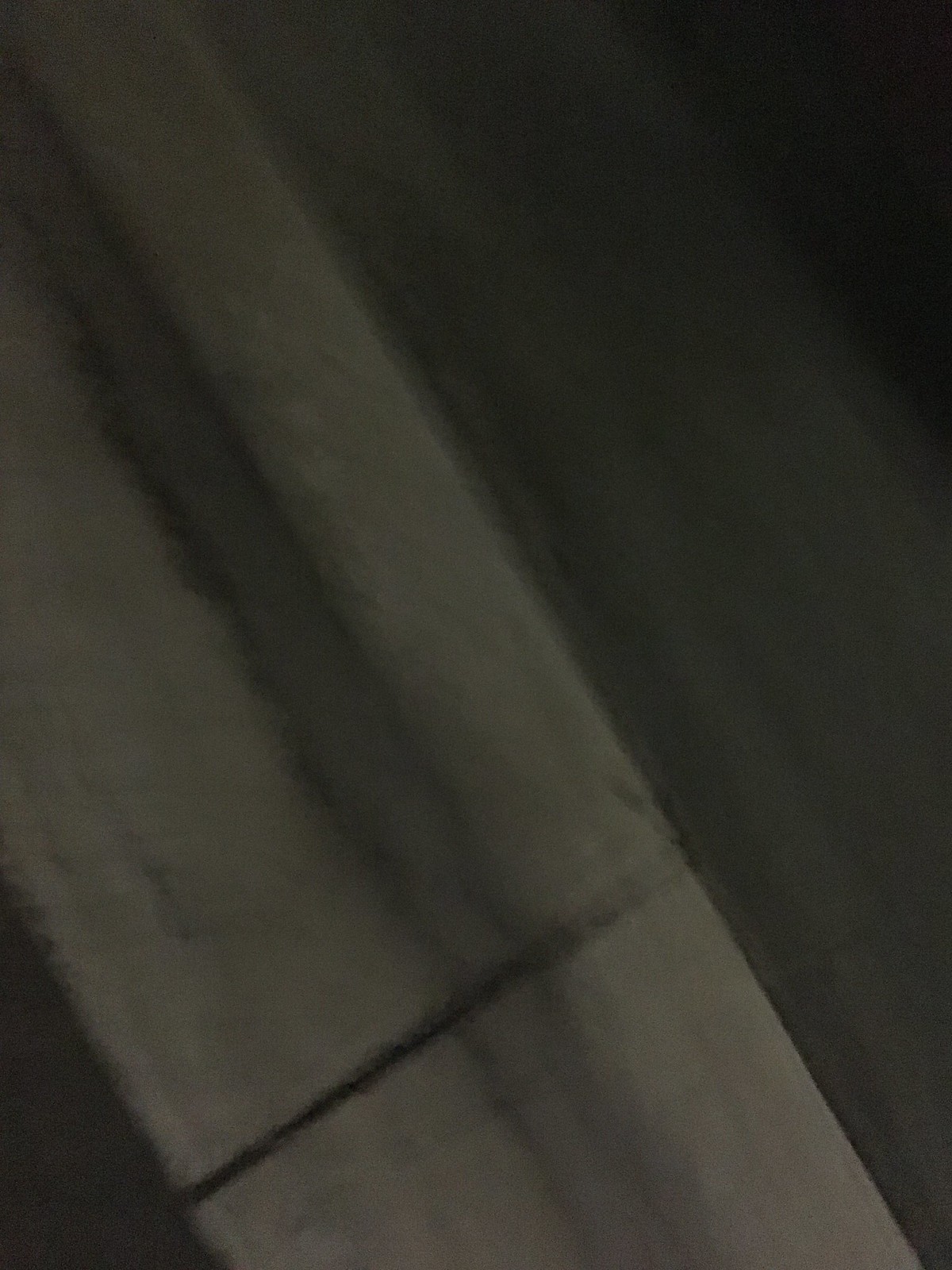The image predominantly features a light gray fabric, likely a curtain given its interweaving pattern and soft appearance. The fabric transitions to a darker shade of gray towards the back, probably due to either lighting or natural color variation. A prominent black horizontal line cuts across the curtain, possibly as part of its design. A lighter rectangular figure slashes diagonally from the upper left to the lower right, intersected by shadows and the black line. The image also includes black spaces in the top right and bottom left corners, adding to the shadowy ambiance. The overall scene lacks clear context, creating an abstract and somewhat mysterious visual.